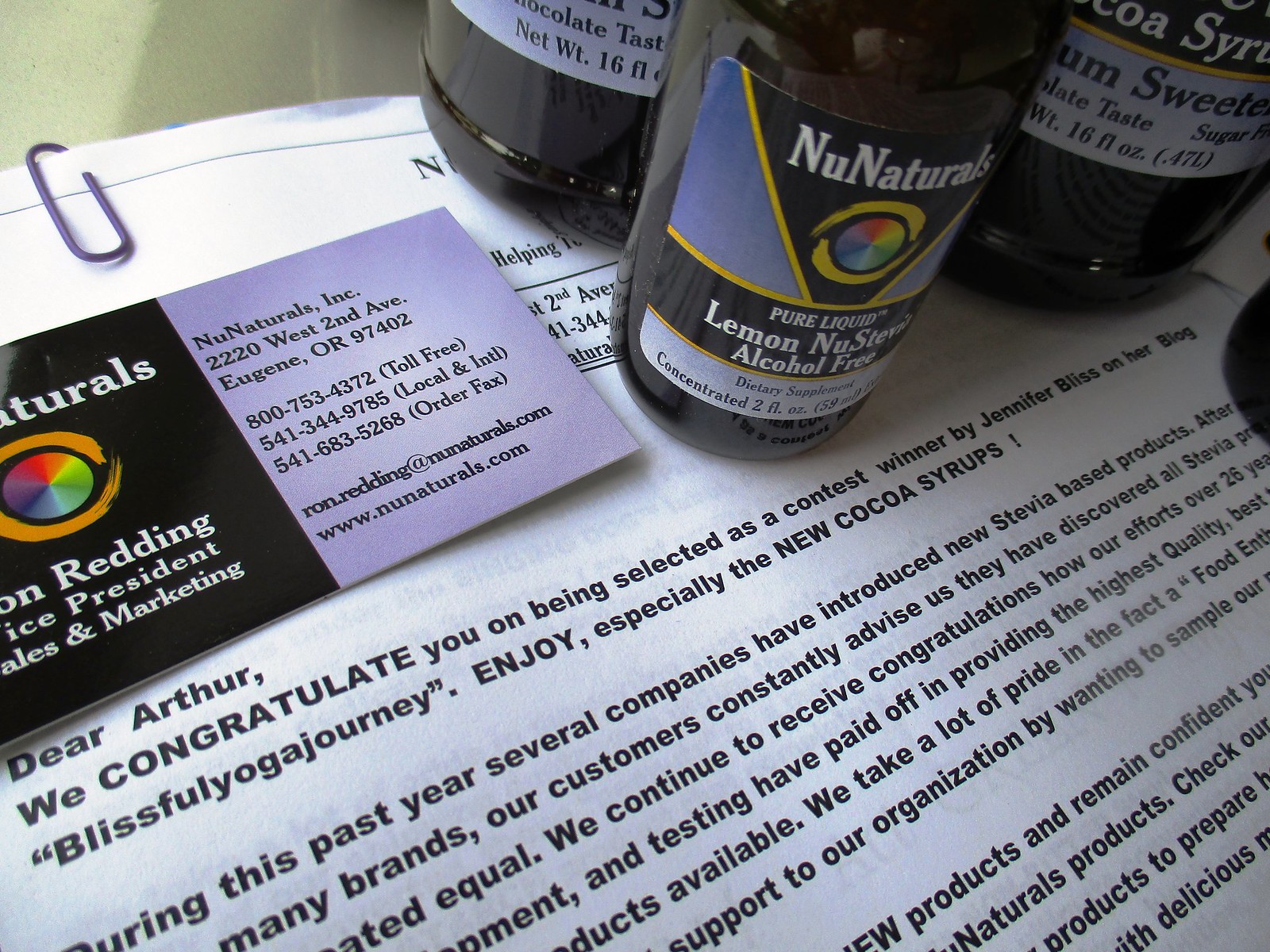The image is a detailed photograph capturing a congratulatory letter addressed to someone named Arthur. The letter, printed on white paper and placed against a gray surface, is partially obstructed by three black-colored supplement bottles labeled with the brand New Naturals. The central design feature on the bottles' labels is a colorful circular logo, and one visible label specifies "Pure Liquid Lemon, Alcohol-Free." Positioned near the top of the paper is a business card from the same company, displaying their address: New Natural Income, 2220 West 2nd Avenue, Eugene, Oregon, 97402. The card also lists several contact numbers: toll-free at 800-753-4272, local and international at 541-344-9785, and an order fax at 541-683-5268, along with an email address and website—www.newnaturals.com. The letter begins with "Dear Arthur, we congratulate you on being selected as a contest winner by Jennifer Bliss on her blog Blissful Yoga Journey," and mentions the inclusion of products like the new cocoa syrup. Additionally, a violet paper clip is visible at the top of the paper.